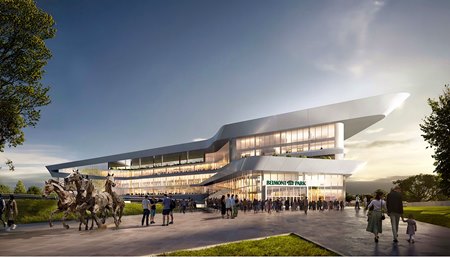This detailed image appears to be a highly realistic architectural rendering, likely not a photograph, of a modern, low-level building with an imposing, contemporary design. The building, potentially a concept for Belmont Park, is characterized by sleek, wide forms made predominantly from steel and glass. The structure, encompassing three to five stories, features a distinctive roof that resembles the hull of a boat. Despite some confusion among viewers, it seems the scene is set during late daylight transitioning to dusk, evident from the illuminated glass interiors contrasting with the dimmer, late-day sky tinged with a mix of white and wispy clouds.

In the scene, there's a bustling sidewalk featuring several pedestrians, including a man, a woman, and a young child holding hands. Notably, there are several horses—three to five—positioned on the lower left side, appearing to run or walk, which seems unusual for this urban setting. This hints at a racetrack environment, further supported by potential signage reading "Belmont Park," reinforcing the equestrian theme. The surroundings include neatly maintained grass patches with edging and a couple of trees—one tall and positioned to the left, another shorter on the right—against a backdrop of a mostly clear sky.